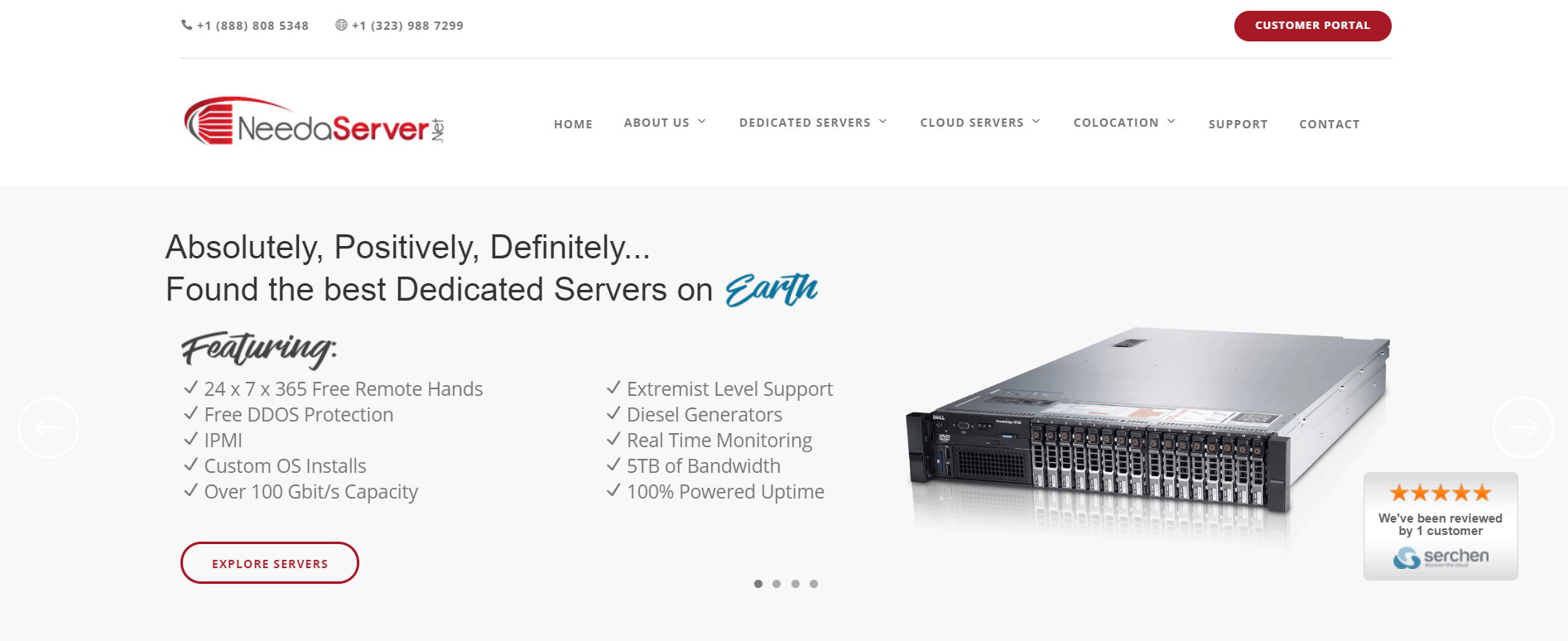This image is a screenshot of a web page with a clean, entirely white background, presented in a slightly wider-than-average landscape style. At the top left corner, there are two phone numbers: "+1-888-808-5348" and "+1-323-988-7299." On the top right corner, there is a prominent red button labeled "Customer Portal."

Immediately below this top section, a thin gray line extends horizontally across the image. Beneath the line, the brand names "Need a Server" and "Need a Server Net" are displayed. To the right, there is a navigation menu with the following labels: "Home," "About Us," "Dedicated Servers," "Cloud Servers," "Co-location," "Support," and "Contact."

Further down, there is a gray horizontal rectangle containing a bold statement: "Absolutely, Positively, Definitely... Found the Best Dedicated Servers on Earth." This declaration is followed by a list of features: "Featuring 24x7x365 Free Remote Hands, Free DDoS Protection, IPMI, Custom OS Installs, Over 100 Gbit/s Capacity, Extremist Level Support, Diesel Generators, Real-Time Monitoring, STB of Bandwidth, 100% Powered Uptime."

At the bottom of the image, a sleek, silver-gray device is partially visible, suggesting advanced technical equipment or a high-tech server. The overall layout emphasizes reliability and superior service in dedicated server hosting.